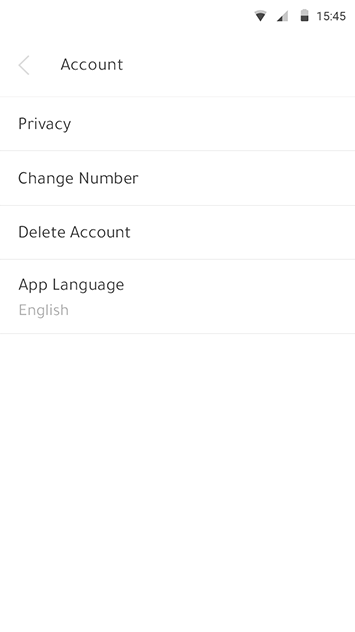The image depicts a smartphone screen with a predominantly white background. At the top, there is a status bar displaying several icons on the right-hand side: Wi-Fi signal, cell signal bars, battery icon at half capacity, and the time, which is 15:45. Below the status bar, the header reads "Account" in black font, accompanied by a backward arrow on the top-left corner. There is a thin gray line dividing the header from the rest of the content.

The main section of the screen is divided into several rows of information, each separated by thin gray lines. The first row contains the word "Privacy" in black font. Following this is the "Change Number" option, also in black. Below that, there is the "Delete Account" option, again in black font with a gray line underneath. The last row features "App Language: English," with "English" in gray font.

The user interface is minimalistic and clean, with most of its elements in black font on a white background. There are no other significant details or graphical elements, emphasizing a straightforward and uncluttered design. The screen seems to pertain to account settings within an application, offering options to change privacy settings, update phone number, delete the account, and select the app language.